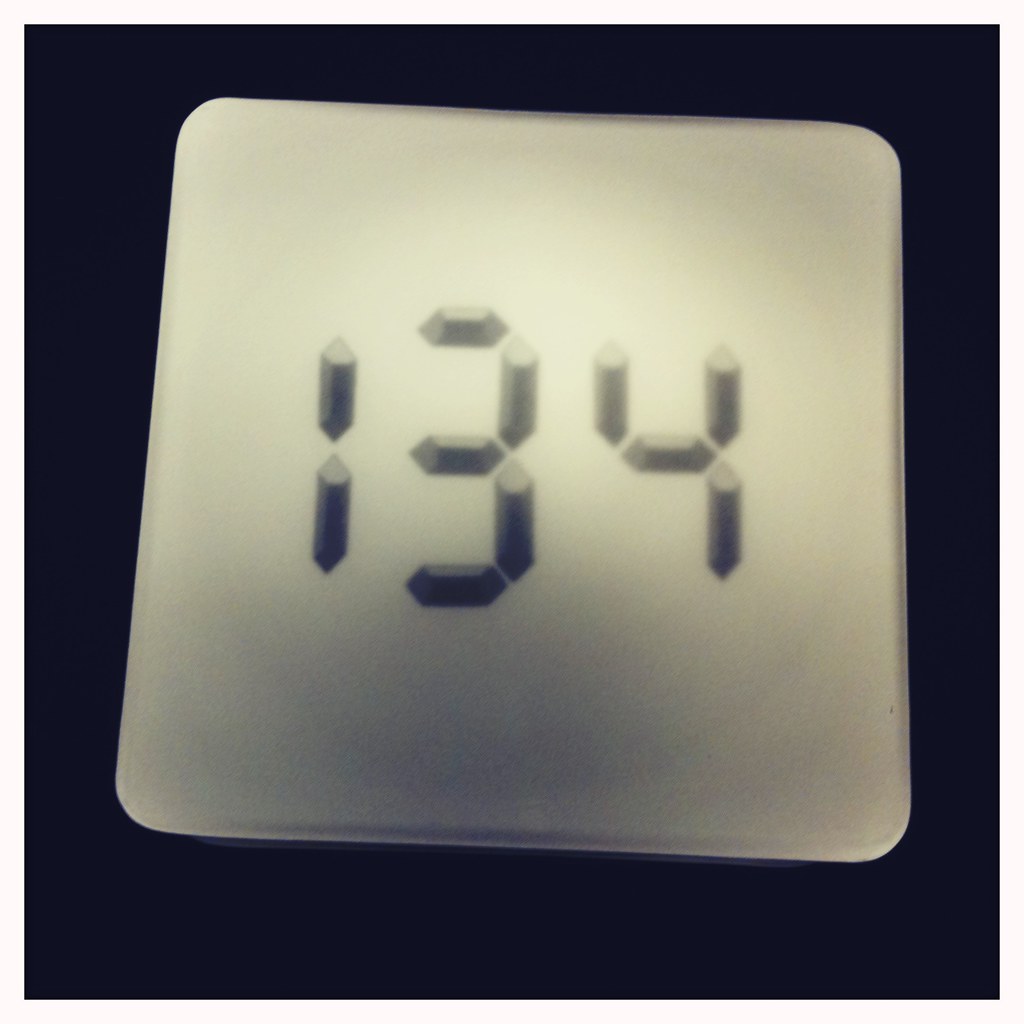The image features an up-close view of a digital display set against a black background. The main focus is a square silver object with slightly curved edges, skewed such that the bottom right corner appears lower than the left. The silver square is bordered by a larger black square frame. In the center of the silver face, the numbers "134" are prominently displayed in a digital-style font, where each digit is comprised of diamond-shaped segments with pointed ends. Notably, the "3" is slightly larger and misaligned compared to the "1" and "4," with its top and bottom segments positioned on higher and lower lines, respectively. The overall impression suggests it could be part of a digital clock, a countdown timer, or a weighing scale, though its exact purpose is ambiguous.